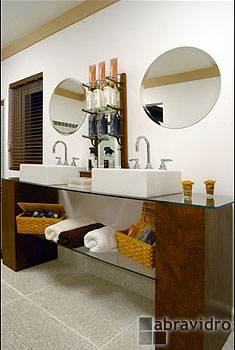This image depicts an elegant bathroom sink vanity setup, likely situated in a high-end resort hotel or luxurious private residence. The white wall, adorned with brown paneling at the top, serves as a backdrop for the refined amenities. The vanity features a his-and-hers configuration, complete with two circular mirrors and two elevated porcelain basins, each paired with sleek silver spigots and separate handles for hot and cold water.

A centrally located rack between the sinks appears to hold various toiletry products, catering to both men and women, though the specific items are not clearly discernible due to the image's small size. These elements are positioned on a glass shelf, which is reinforced with wooden supports on each side.

Below the main vanity surface, another glass shelf displays neatly rolled towels alongside two wicker baskets, presumably containing additional toiletries and accessories. The gray-tiled floor complements the overall sophisticated aesthetic.

A window with brown pull shutters, absent of any curtain, allows natural light into the space, enhancing the warm and inviting atmosphere. The image also features a watermark from a company named either AbraVidro or LabraVidro, depending on the interpretation of the logo's design.